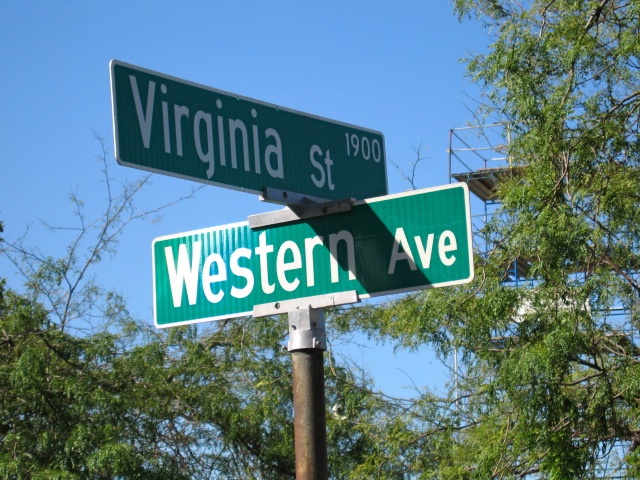In the image, there is a close-up of two intersecting street signs mounted on a dark, silver metal post that appears rusted at the bottom. The sign at the top is green with white trim and prominently displays "Virginia Street" in large letters, with the number "1900" in the top right corner. The intersecting sign, oriented in a different direction, is similarly green with white trim and reads "Western Avenue." The view of the signpost is cut off at the bottom. In the background, lush trees extend to the left, center, and right, while a clear blue sky without clouds provides a serene backdrop. Additional structures visible in the distance include tall metal rafters with multiple levels, suggesting they might be used for constructing billboards.